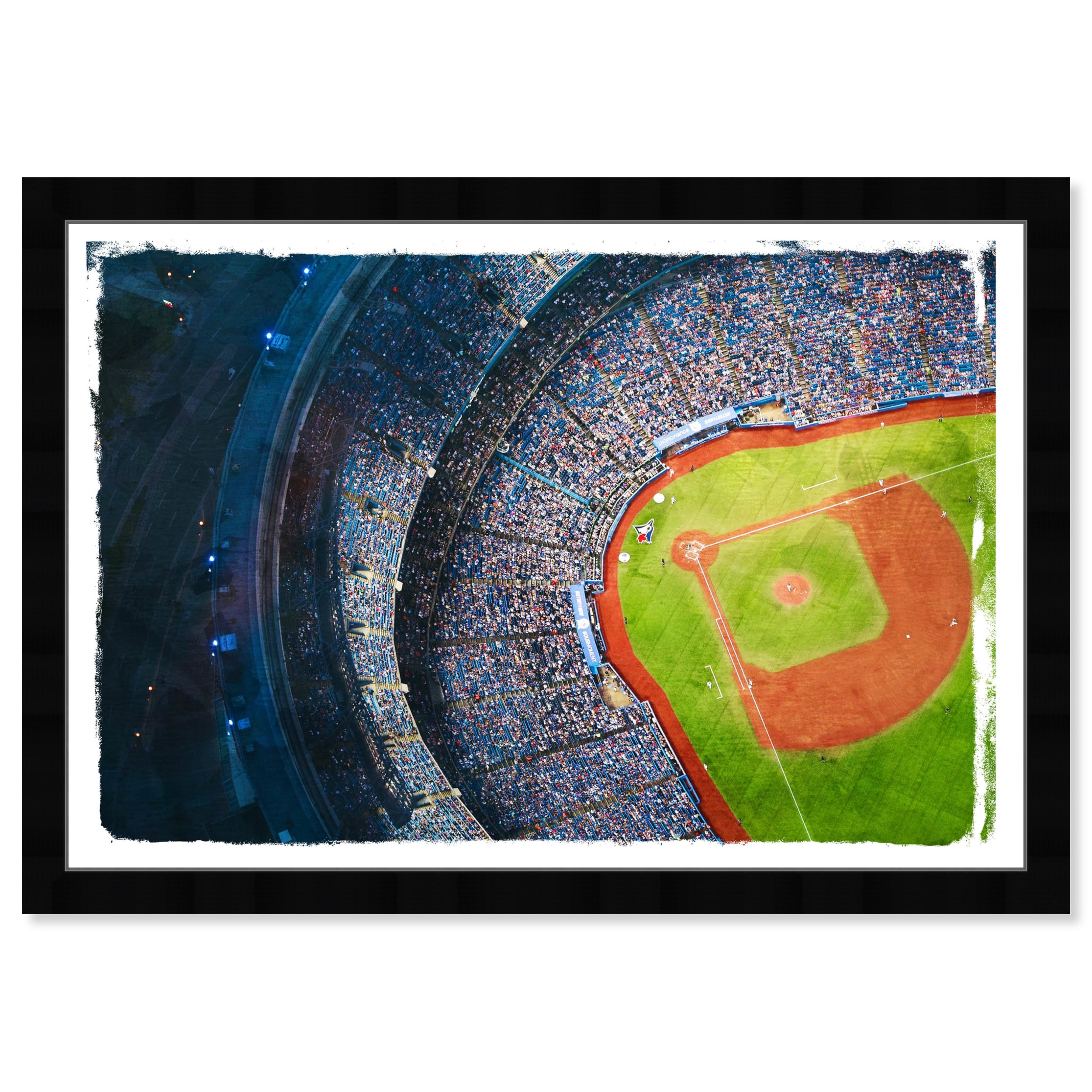The image is a rectangular framed art print, measuring approximately five inches wide and three inches high. It features a narrow black frame, about a quarter of an inch wide, surrounding a thin, dark gray pinstripe line. Inside this, the printed image is bordered by a white margin with slightly ragged edges.

The central image is an aerial view of a baseball stadium, predominantly focused on the lower right section. Here, a vibrant green baseball field is outlined with brown dirt, showcasing the distinct shape of the diamond. The field includes white-painted bases, the pitcher's mound, and the catcher's and batter's areas, with a Blue Jay logo visible behind home plate. The stadium appears to be packed with spectators dressed mainly in blue and white, indicating a lively, night-time game as only the stadium is illuminated against a darker outer environment.

The seating sections curve around the top and left sides of the image, packed with multiple levels of fans. At the edges of the stadium, there are indications of gray streets with white lines, further emphasizing the bustling atmosphere surrounding the baseball game.